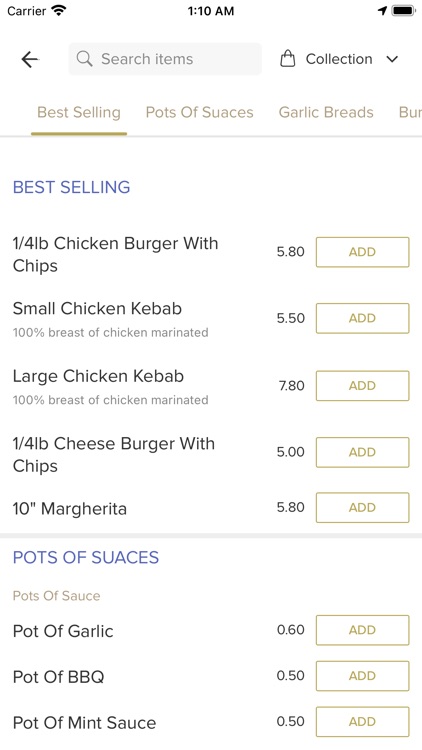The image appears to be a screenshot or a page from a food delivery app, likely displaying menu items and prices. At the top, it features a search bar with the label "Carrier, 110 AM" and an arrow pointing to the left suggesting a navigation option.

Below the search bar, there's a section titled "Collection, Best Selling Pots of Sauces, Garlic Breads," hinting at curated categories of popular items available for purchase. 

Under the "Best Selling" section, a variety of mouth-watering items are listed with their prices:
- A Quarter Pound Chicken Burger with Chips for $5.80.
- A Small Chicken Kebab priced at $5.50.
- A Large Chicken Kebab for $7.80.
- A Quarter Pound Cheeseburger with Chips for $5.00.
- A 10-inch Margarita Pizza available at a bargain price of $5.80.

Further down, there's a distinct line separating the main dishes from the condiments section. This part showcases a variety of sauces:
- Pot of Garlic for $0.60.
- Pot of Barbecue Sauce for $0.50.
- Pot of Mint Sauce also for $0.50.

Overall, the menu flaunts a selection of appetizing dishes and condiments at very reasonable prices.